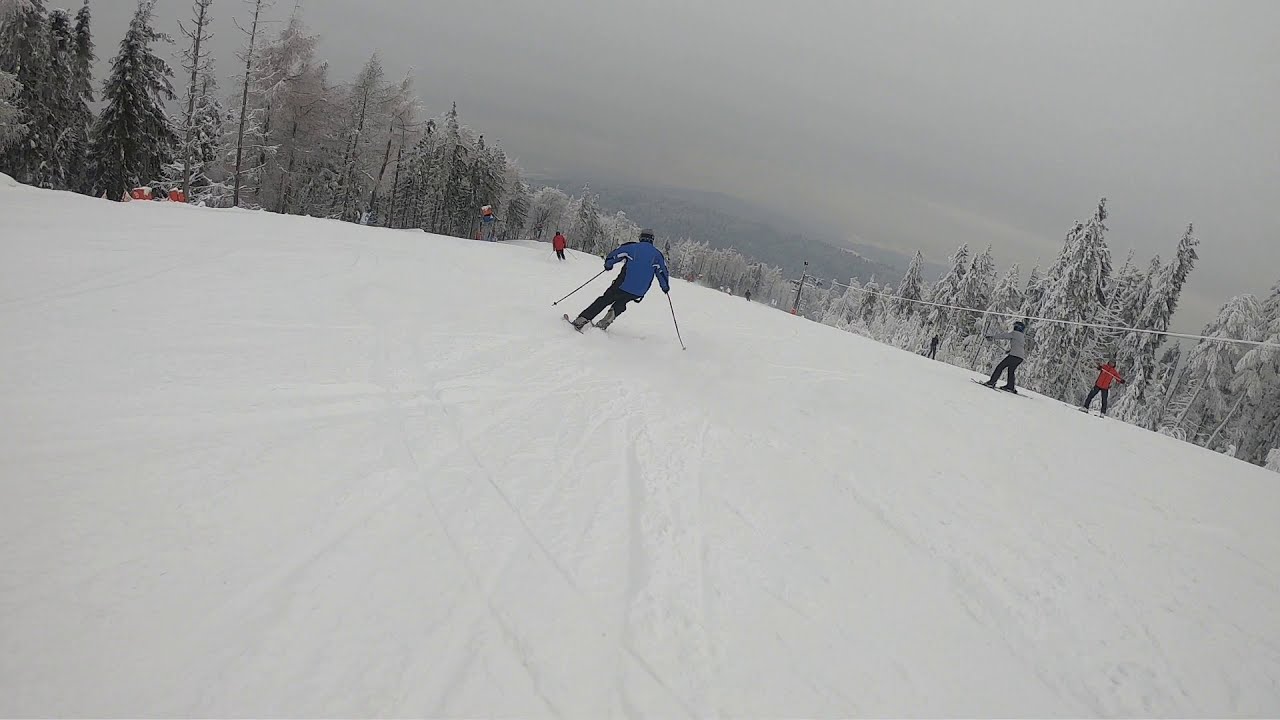In this photograph of a winter ski scene, the ground is completely covered in pristine white snow, punctuated by narrow ski trails left by previous skiers. The foreground features a skier dressed in a blue jacket and black pants, holding ski poles as he glides across the flat snow-covered terrain. Flanking the snowy path are dense evergreen trees, their branches heavily laden with white powder. Grayish clouds fill the sky, creating an overcast and somewhat hazy backdrop that envelops the distant mountainous area. Additional skiers appear in the image: one in a gray jacket and black pants to the right, another in a red jacket and black pants further into the scene, and a tiny figure in red and black off to the left. Overhead, a wire indicative of a ski resort hinting at the remoteness of this winter wonderland. Despite the serene and predominantly white landscape, the ski tracks indicate a well-frequented location.